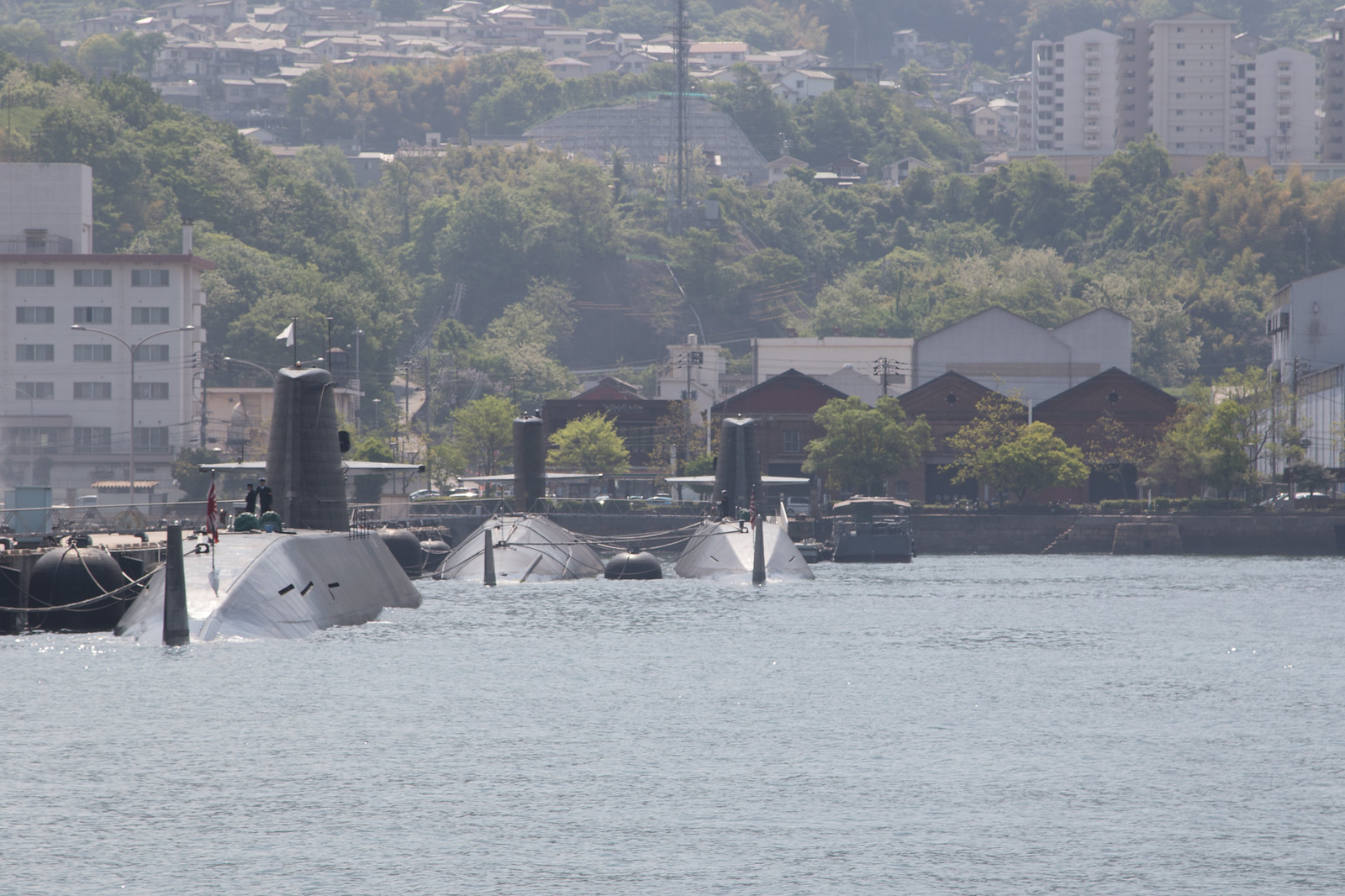The photograph captures a vivid lakeside scene with an intriguing mix of urban and maritime elements. In the foreground, the dark, slightly choppy water of the lake spans almost the entire bottom half of the image. Prominently, three silver, partially submerged submarines are docked at a pier that stretches from the right towards the center. Each submarine features a bulbous, domed top with a vertical extension or tower emerging from the center, resembling smokestacks, and adorned with various flags. The shoreline is lined with small, uniform architectural structures, visible only by their roofs. In the background, a series of identical brick warehouse buildings stand along the docks, while beyond them, a cityscape of apartment buildings and rooftops rises against a backdrop of green trees on a hill, suggesting a hilly terrain. The overall scene blends the serene natural elements with the structured, industrial harbor, creating a captivating contrast.